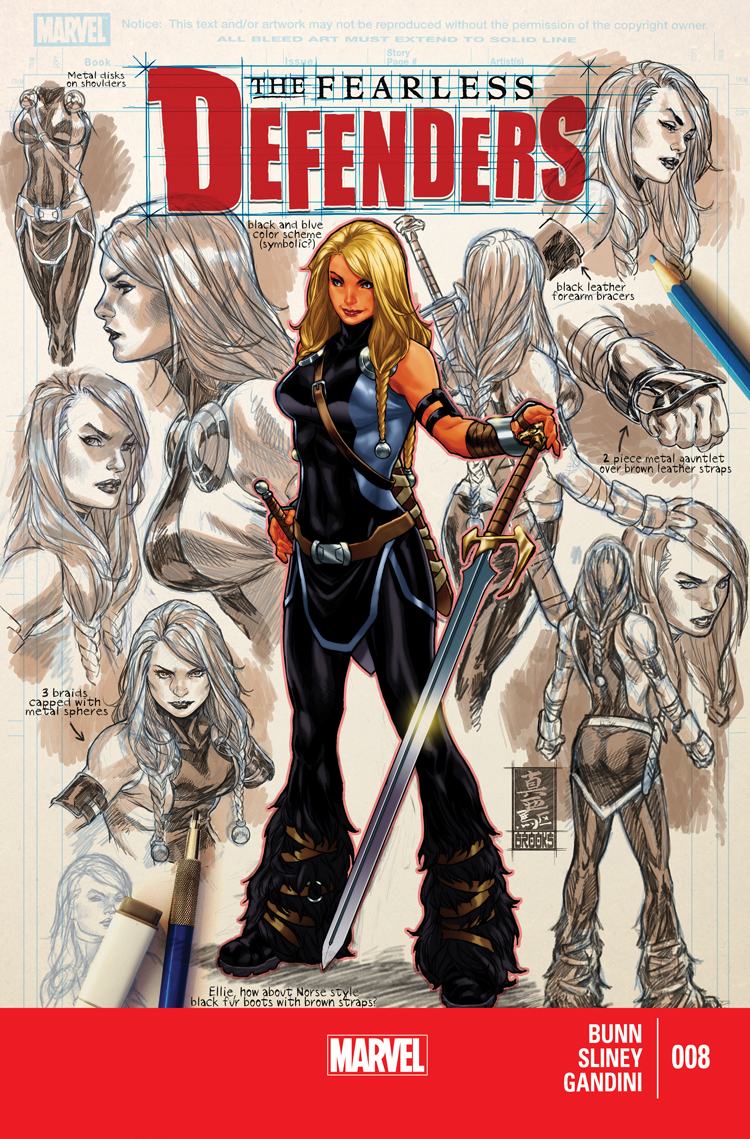The comic book cover features an eggshell off-white background with the Marvel logo prominently displayed in the top left corner. Below the logo, "The Fearless Defenders" is written, with "Fearless" in black and "Defenders" in bold red letters outlined in blue and black. The cover is adorned with star shapes in each corner. At the center, a fully-colored illustration of a Caucasian woman with long blonde hair is depicted. She wears a tight-fitting black bodysuit with blue trim and has black pants that end in fur-bound straps around her boots. She holds a large, ornate sword with a brown handle and shiny silver blade, while her other hand grips a dagger. Surrounding the main image are multiple black-and-white sketches of the same character, showing various facial expressions and angles. At the bottom, a red band displays the text "Marvel" in white and alongside, the names "Bun, Sliny, Gandini 008" are listed in the bottom right corner.